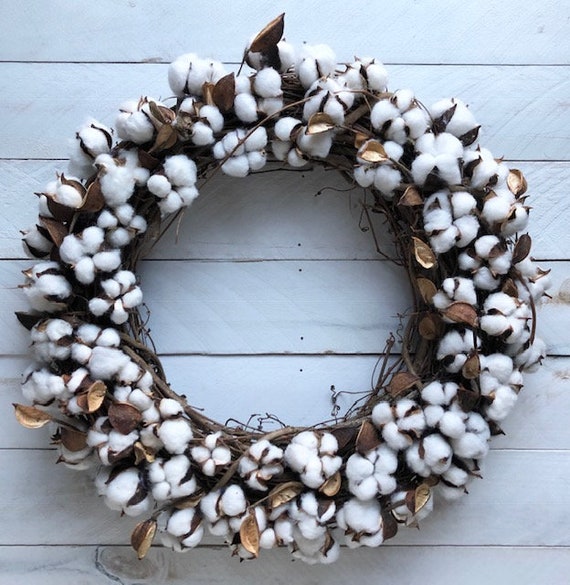This image captures a small, round wreath boasting a charming, rustic, country-like style. Crafted from small, wooden twigs and branches, the wreath is adorned with delicate, white blooms resembling cotton flowers or possibly dogwood. These blooms, reminiscent of little cotton balls, are scattered uniformly across the wreath, adding a whimsical touch. The wreath also features gold leaves extending from its edges, adding a touch of elegance amidst the natural textures. The base color palette comprises primarily of the brown from the twigs and the snowy white from the cotton-like flowers. This beautifully messy, yet intentionally designed wreath is mounted against a distressed, off-white wooden backdrop, which enhances its rustic appeal and brings out the earthy elements of the decoration.